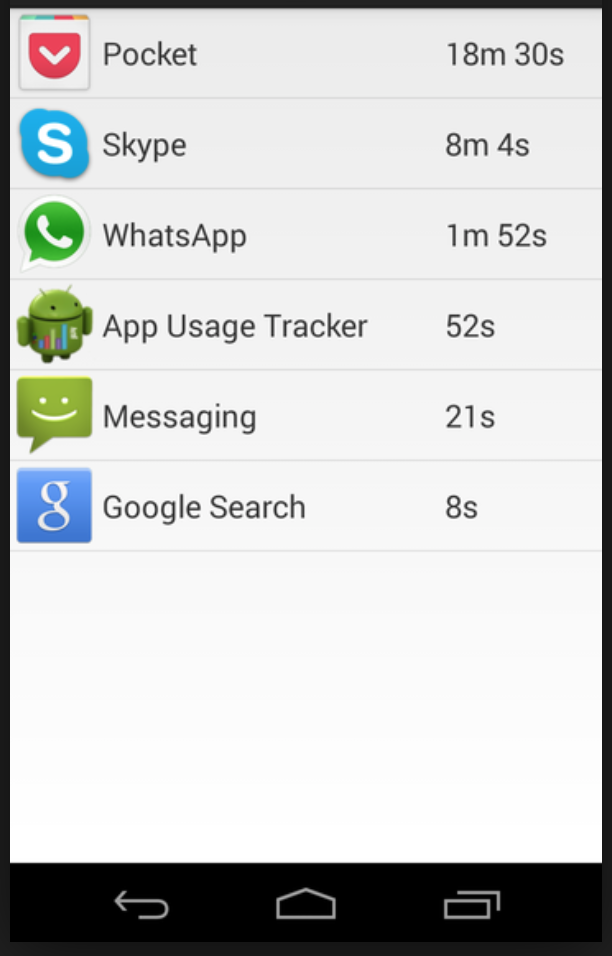This screenshot captures a detailed list of application usage on a phone, highlighting the duration each app has been used. 

The first entry is the "Pocket" app, whose icon resembles a red pocket with colorful accents at the top and a downward-pointing white arrow. It indicates 18 minutes and 30 seconds of usage. 

Next is "Skype," denoted by a blue circle with an "S" in the center, showing a usage time of 8 minutes and 4 seconds.

Following Skype is "WhatsApp," represented by a green speech bubble containing a white phone icon, reflecting a usage duration of 1 minute and 52 seconds.

The "App Usage Tracker" is highlighted with an icon of an Android robot displaying bar graphs on its torso, signifying 52 seconds of use.

"Messaging" is showcased with a green, rectangular speech bubble icon featuring a white smiley face, indicating 21 seconds of activity.

Lastly, "Google Search" is marked by a blue square containing a white "G," registering 8 seconds of usage.